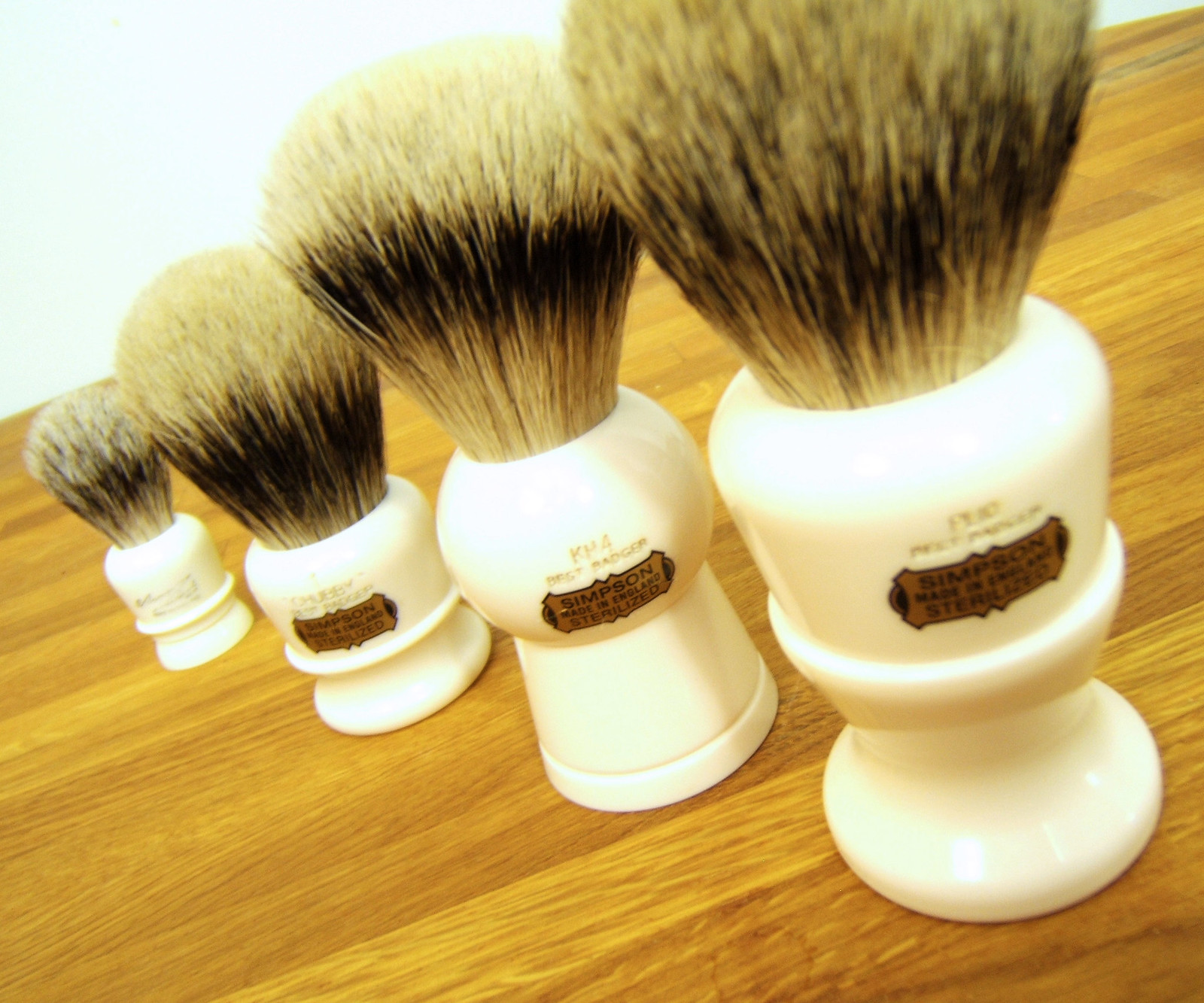This up-close photograph showcases a set of four shaving brushes, each meticulously arranged diagonally atop a brown and yellow wooden surface. The brushes, varying slightly in size with the largest on the bottom right corner and the smallest progressing toward the middle left corner, all share identical designs. Each brush features a circular white handle base that tapers upward, widening into a cylindrical section that prominently displays a gold sticker with black lettering. The sticker includes the brand name "Simpson", "Made in England", and "Sterilised". Additionally, there's an inscription "KH4 Best Badger" in gold. The bristles of the brushes are tri-colored, transitioning from yellow at the base to a dark brown center, and fading back to a yellow hue at the tips. The meticulous details, consistent color scheme, and branding on each brush suggest a high-quality set designed for a refined shaving experience, all uniformly aligned to emphasize symmetry and elegance.